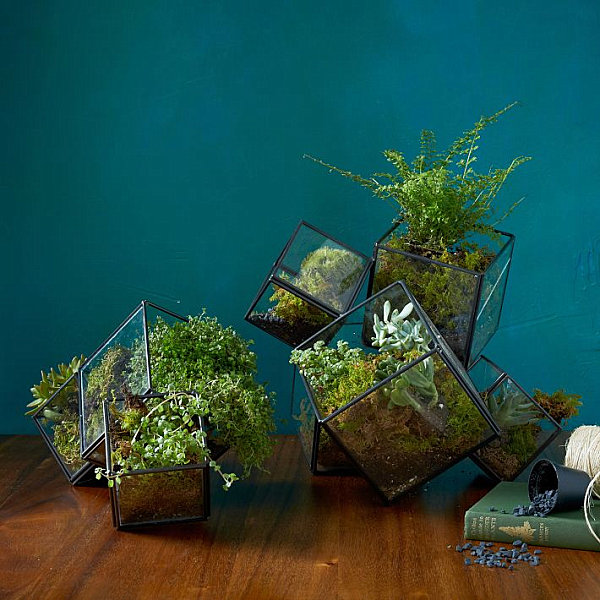In the photograph, there's an indoor still life scene with a bluish-green background, showcasing a collection of six square glass terrariums with black frames, artfully arranged on a brown wooden table. These glass containers, each housing an assortment of green plants including succulents and a specific cortis plant, are intentionally tilted at various angles, creating a dynamic and artistic composition. Inside the terrariums, the bases appear mossy, adding a lush, natural texture. Behind some of the containers, taller plants are visible, contributing to the layered visual depth. 

On the right side of the table, a hard-covered green book lies tipped over, next to a blue plastic container, from which tiny decorative blue stones have spilled out, scattering across the wooden surface. Additionally, there is a reel of tan-colored twine placed further back on the table. The overall color palette of the image includes shades of green, blue, brown, black, gray, and white, evoking a tranquil and earthy atmosphere. The photograph is square-shaped, emphasizing its balanced and composed aesthetic.